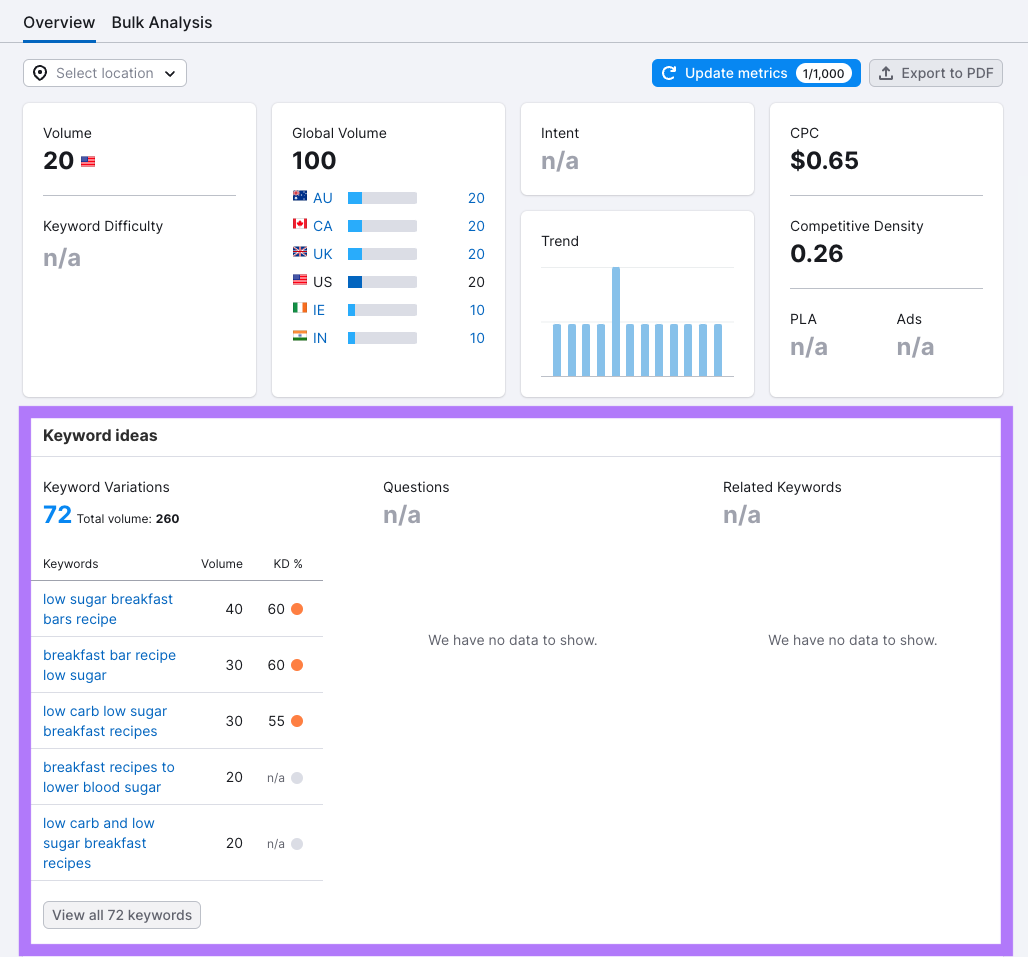The image displays a detailed analytical interface on a gray background, showcasing a variety of charts and data points. In the upper left-hand corner, "Overview and Bulk Analysis" is prominently printed in black, with "Overview" underlined in blue. Below this, there is a "Set Location" option accompanied by a drop-down menu.

On the right-hand side, the section reads "Update Metrics: 1 of 1,000," featuring a refresh icon. The "Export to PDF" option is grayed out. A white box labeled "Volume 20" is marked with an American flag. Below these metrics, several data points are listed, including "Keyword Difficulty: n/a," "Global Volume: 100" (distributed as 20 AU, 20 CA, 20 UK, 20 US, 10 IE, and 10 IN), "Intent: n/a," and "Trend," which is represented by a blue chart. The trend chart shows consistent heights for the first four segments, a spike doubling the height in the fifth segment, and a return to the original height for the remaining segments.

Further metrics displayed include "CPC: $0.65," "Competitive Density: 0.26," "PLA: n/a," "Ads: n/a," and "Keyword Ideas" broken down into "Keyword Variations: 72" and "Total Volume: 260." The "Questions" and "Related Keywords" sections are marked as "n/a."

A list of specific keywords follows, including "Low Sugar Breakfast Bars Recipe," "Breakfast Bar Recipe," "Low Sugar," "Low Carb," "Low Sugar Breakfast Recipes," "Breakfast Recipes to Lower Blood Sugar," and "Low Carb, Low Sugar Breakfast Recipes." A prompt to "View all 72 keywords" is included, with the "Keywords Idea" section highlighted by a purple border.